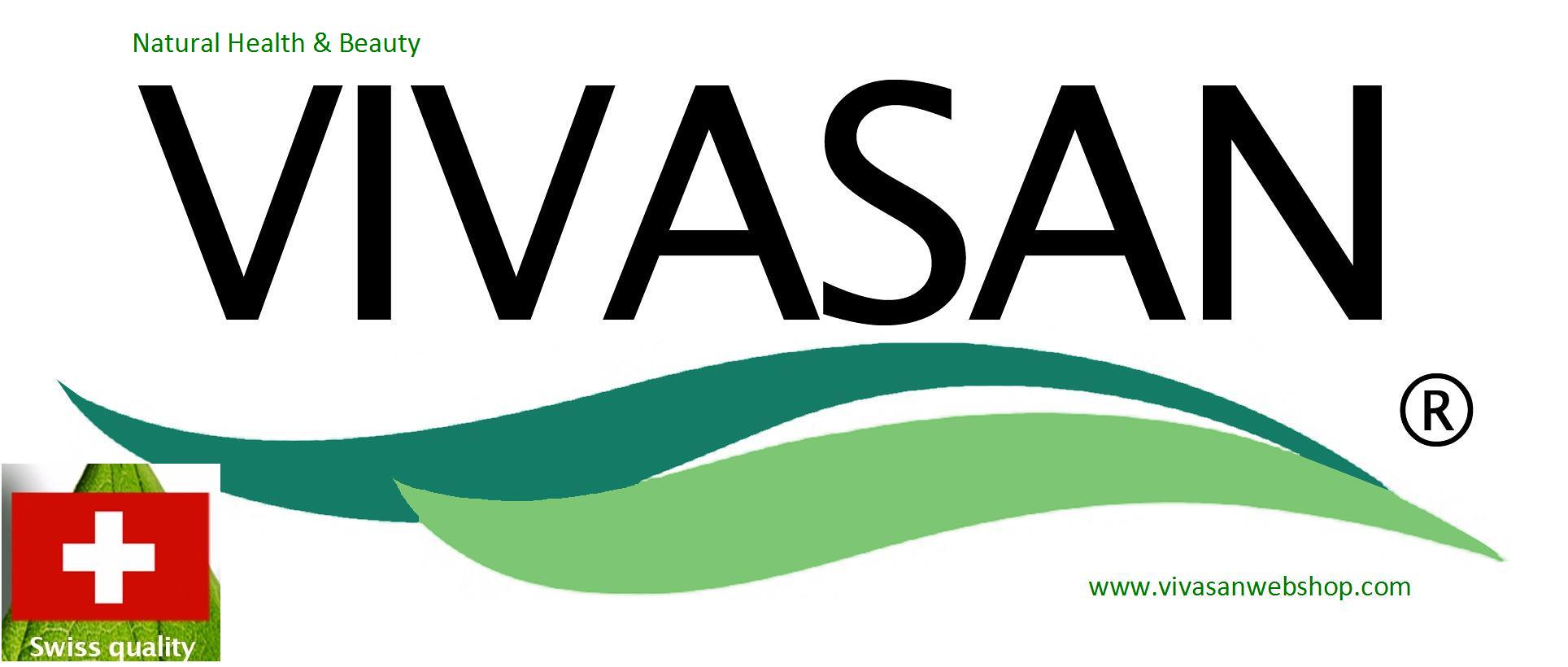This image is a detailed advertisement for the company Vivasan, emphasizing natural health and beauty products. The primary focus of the image is the word "Vivasan" prominently displayed at the top in bold black letters, accompanied by a small trademark symbol (R) to its right. Directly beneath the company name are two wavy designs that resemble leaves—one in a lighter green and the other in a darker green—adding a natural aesthetic to the ad. Below these designs, the website address "www.vivasanwebshop.com" is clearly listed. On the bottom left corner of the image sits the Swiss quality logo, which features a red square with a white cross at its center, further highlighted by a surrounding green, red, and white circular design. The logo signifies the Swiss origin and quality of Vivasan's products.